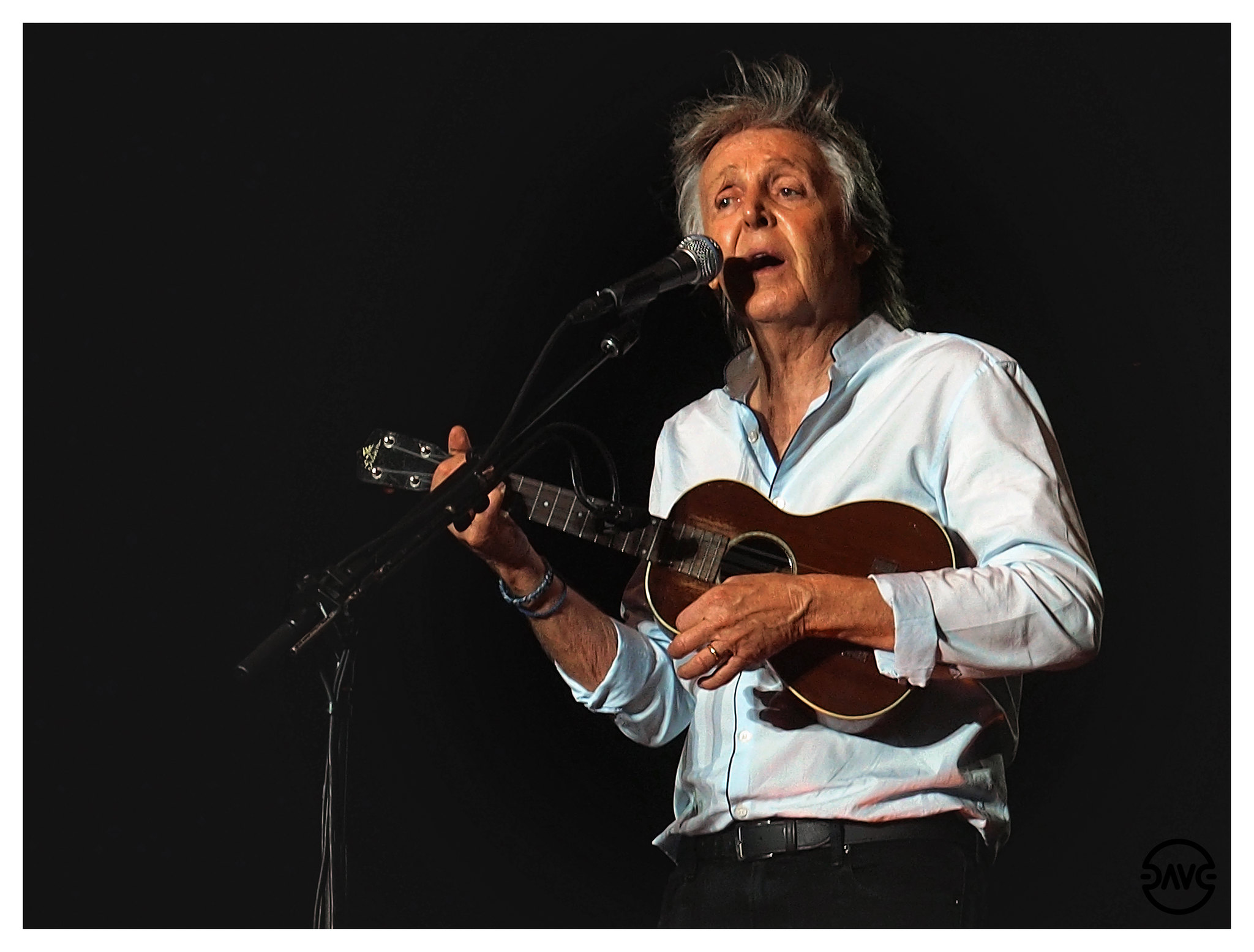In this recent photograph, Paul McCartney is captured mid-performance at a concert. He is playing a small guitar or ukulele-like instrument, which he holds with both arms. His left arm, bent at a 45 to 90-degree angle, strums the strings. A large black microphone stand extends out of the frame, reaching up for about three feet with a microphone attached. Dressed in a blue dress shirt with the top buttons undone, McCartney appears relaxed and focused. He is clean-shaven with white, longish hair that cascades to his shoulders in the back and is styled reminiscent of a "Flock of Seagulls" look in the front. He accessorizes with a black belt and black pants, which appear to be jeans, though the precise style is indistinguishable due to the framing. A wedding ring adorns his left ring finger, accompanied by bracelets or a watch on his left wrist. The brown guitar shows some wear near the top of the fretboard, adding a touch of character to the image. The backdrop is completely black, suggesting the concert is taking place at nighttime.